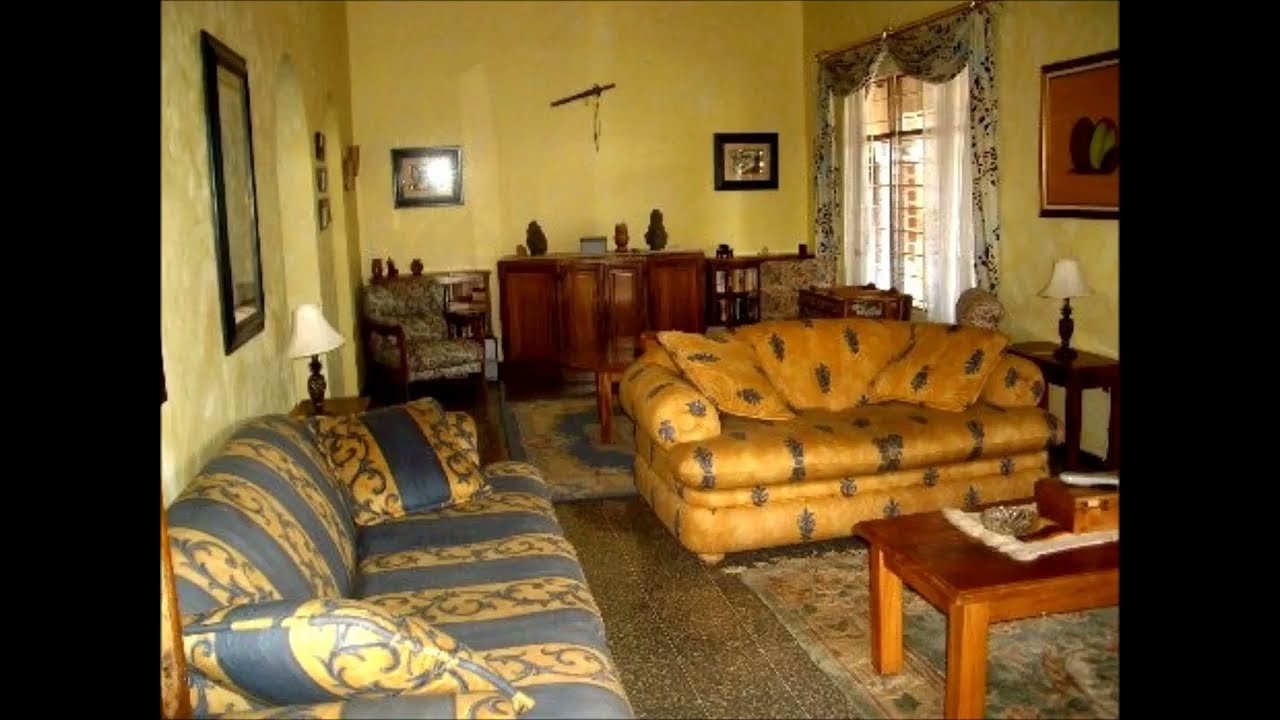This image captures a cozy, small home, characterized by a reddish-pink tiled roof and white exterior walls. The scene appears to be in what might be a backyard or outdoor living area. A notable feature is a bar area on the right with four brown stools set beneath the roof, giving it an indoor-outdoor ambiance. On the left side, there's a window adorned with white curtains. In front of the house, a small cement table is flanked by three cement benches, providing a quaint seating arrangement. Surrounding the house are lush sections of grass filled with small plants, and the ground itself seems to consist primarily of clean clay or dirt. Elegant brick posts support the structure, with vibrant yellow flowers climbing up them. Additionally, a palm tree stands prominently in front of the door, accompanied by an array of flowers in shades of pink, yellow, and red. The sky appears white, allowing the vivid greenery and colorful flora to stand out, giving the home a welcoming and picturesque atmosphere.